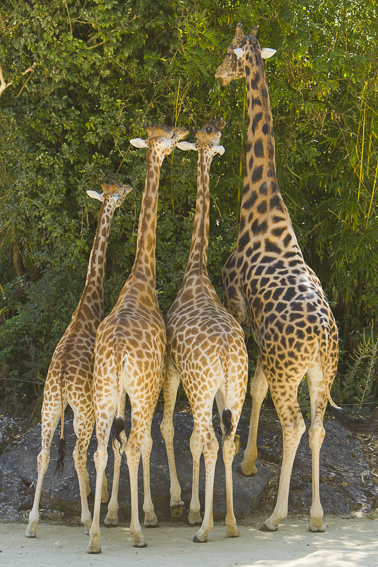The image displays the back view of four giraffes standing in an outdoor setting arranged from shortest to tallest from left to right. The tallest giraffe, presumably the parent, is on the far right and has one foot on a brownish to grayish rock, allowing it to reach the leaves of a tall tree in front of them. This giraffe has darker spots compared to the others. The three smaller giraffes, with lighter spots, are on the left, middle, and right positions below the tallest one, gazing upwards, seemingly unable to reach the leaves. The scene is set on a light brown or beige concrete ground, and the focus is so close that little else is visible in the frame.